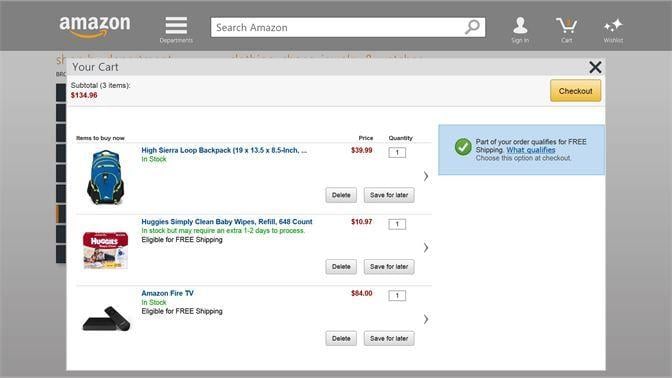This image is a detailed screenshot of an Amazon cart, captured in color. Dominating the top of the image is a dark gray banner bar featuring the Amazon logo positioned on the left side. To the right of the logo is a "Departments" button, followed by a search bar, and icons labeled "Sign In," "Cart," and "Wish List."

Beneath this bar, the screen displays the user's cart section. A gray banner at the top of this section reads "Your Cart" on the left and has an "X" for closing the cart on the right. The background shifts to white, displaying a subtotal for three items amounting to $134.96. A yellow "Proceed to Checkout" button is located on the left side, alongside the subtotal text, and to its right, a summary column.

The first item in the cart is a "High Sierra Loop Backpack," priced at $39.99 and listed in stock with a quantity of one. The second item is a 648-count box of "Huggies Simply Clean Baby Wipes," priced at $10.97. It is also in stock but with a note indicating an extra processing time of one to two days. The third item is an "Amazon Fire TV," priced at $84.00, shown as in stock and eligible for free shipping.

To the right of the item list, a blue rectangular box provides a shipping notice, indicating, "Part of your order qualifies for free shipping. What qualifies? Choose this option at checkout." This message suggests possible savings for the customer if they select the appropriate shipping option during checkout.